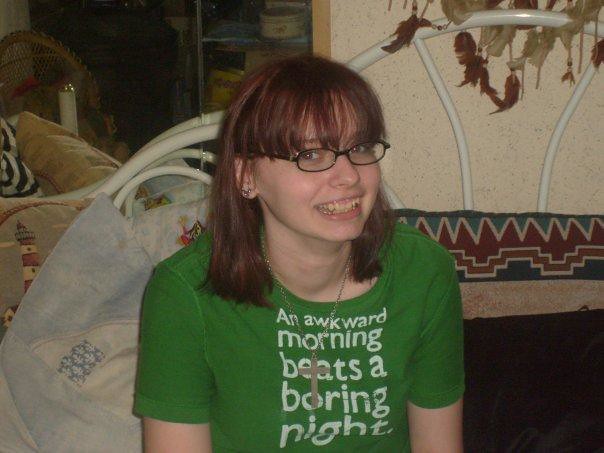In the photograph, a young woman, possibly in her late teens or early twenties, is seated on a piece of furniture that resembles a daybed or futon with a white metal frame. She has short, reddish-brown hair with bangs and is wearing dark-framed glasses, earrings, and a large silver cross necklace. She is dressed in a green t-shirt with the white text "An Awkward Morning Beats a Boring Night." Despite her wide, toothy smile, there is an air of slight discomfort. 

Behind her, there is a cluttered background featuring various elements. To her left, there is a wicker chair and a storage cupboard, while directly behind her head is a shelf. A blue and white pillow and another pillow with a lighthouse design are positioned behind her. To her right, more of the daybed frame and additional pillows are visible, along with the bottom of what looks like a dreamcatcher hanging in the upper right corner. This detailed and eclectic scene suggests a cozy, albeit cluttered, environment in what could be a living room or a similarly multifunctional space.